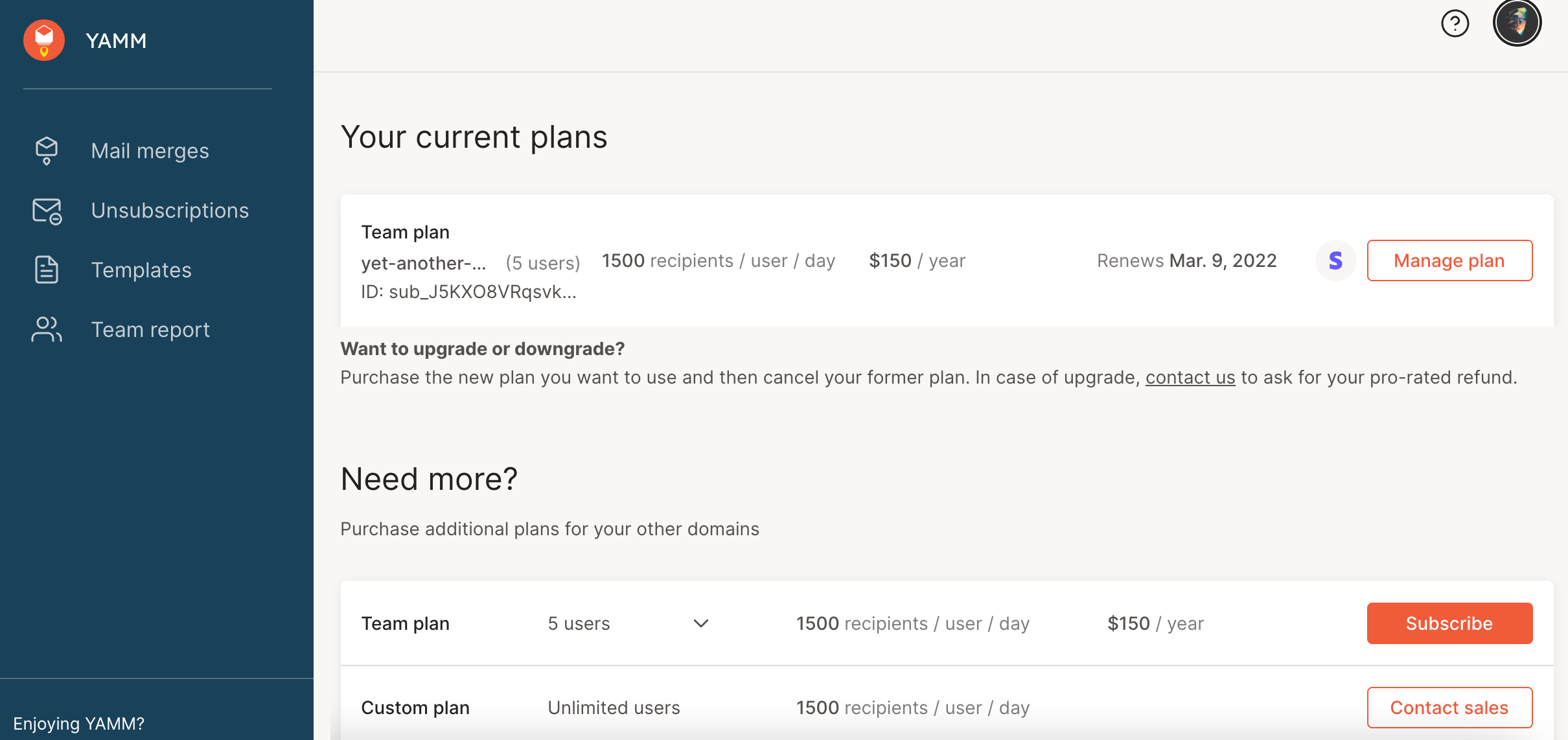A screenshot with a gray background and a blue section to the left. The blue section prominently features the acronym "YAMM" in white, all capital letters. Below it, there's a list of options including "Mail merges," "Unsubscriptions," "Templates," and "Team report."

The screenshot details the "Your current plan" section, indicating it is a "Team Plan" (both terms are in bold). The plan covers "Yet Another" (5 users), allowing 1,500 recipients per user per day. The cost is $150 per year, with "$150" in bold. The renewal date is shown in bold as "Mar. 9, 2022."

There is a blue circle with a dollar sign and an orange rectangle that says "Manage Plan." Additional text provides an ID number and instructions for upgrading or downgrading the plan. It advises purchasing the new plan you desire and then cancelling the previous one. It also notes that, in case of an upgrade, you should contact support (the word "contact" is underlined) to request a prorated refund.